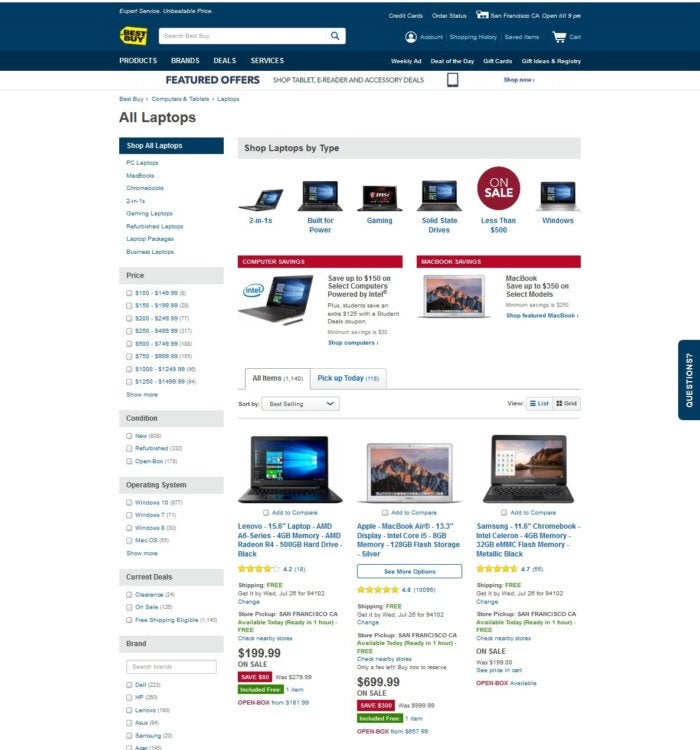The website displayed is from Best Buy, dominated by a recognizable yellow label with "Best Buy" written in black. This logo is situated on a blue navigation bar that features a white search bar prominently in the center. The navigation bar includes categories such as Products, Brands, Deals, and Services. On the right side of the bar, additional options like Weekly Ad, Deal of the Day, Gift Cards, Gift Ideas, Registry, and a shopping cart icon are present.

Scrolling down reveals featured offers, including sections like "Shop Tablet, E-Reader, and Accessory Deals." Users have the option to shop via phone or click "Shop Now." Next, there's a detailed section for laptops. "All Laptops" is highlighted in a blue banner, and within this section, "Shop All Laptops" is prominently displayed on a blue illuminated button. Below, in a gray bar, the site invites users to "Shop Laptops by Type," showcasing various categories of laptops.

Highlighted items feature red circle badges marked "On Sale" with prices below $500. The section contains multiple images of laptops, with two red informational bars that are too small to read. There’s also a "Pick Up Today" option highlighted in blue, and beneath it, options to sort listings, view different lists, and additional gray text which is unreadable due to its small size.

Further into the selection of laptops, each item is accompanied by a star rating and an 'Add to Cart' option. Prices range from $1.99 for an item on sale, up to $699.99 and $999.99. Some items are highlighted as "On Sale" with accompanying red or green buttons, except for one open box item which lacks these buttons. On the left sidebar, filtering options include Price, Condition, Operating System, Current Deals, and Brand.